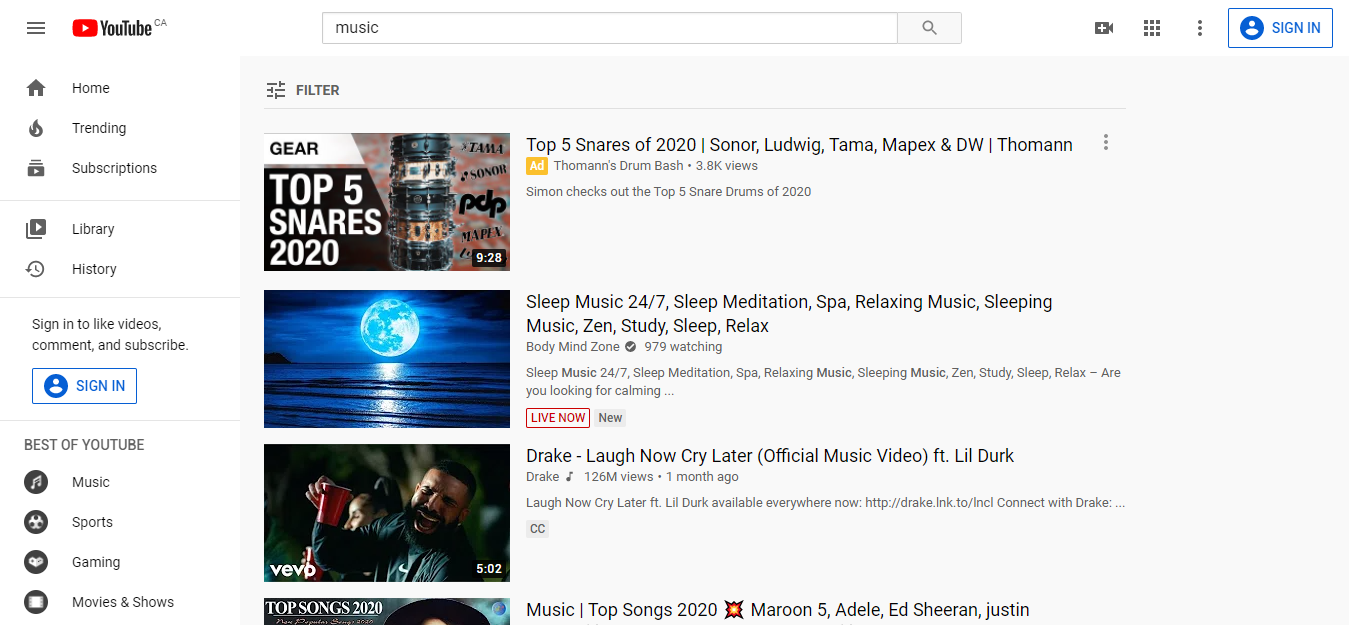In this screenshot of a YouTube search for "music," the top results display a variety of content. The first video is an advertisement titled "Top Five Snares of 2020" by Sonor and Ludwig, identified by an orange ad box. The video is 9 minutes and 28 seconds long, featuring Simon's review of the top five snare drums of the year. The second result is a live stream labeled "Sleep Music," which loops relaxing music to aid in sleep and relaxation. The third video is the official music video for "Laugh Now Cry Later" by Drake, with over 100 million views, uploaded one month ago, and includes a link to purchase the digital album. The fourth video, partially obscured at the top, appears to be a compilation titled "Music Top Songs 2020," featuring artists like Maroon 5, Adele, Ed Sheeran, and Justin Bieber.

To the right of the search results, there is a video tutorial on creating and uploading YouTube videos. Above this, there are icons including a grid of nine squares for accessing other YouTube apps, three dots for format options, and a sign-in option. On the left-hand sidebar, underneath the main YouTube logo, are links to Home, Trending, Subscriptions, Library, History, and "Best of YouTube" categories, which include sections for Music, Sports, Gaming, and Movies & Shows.